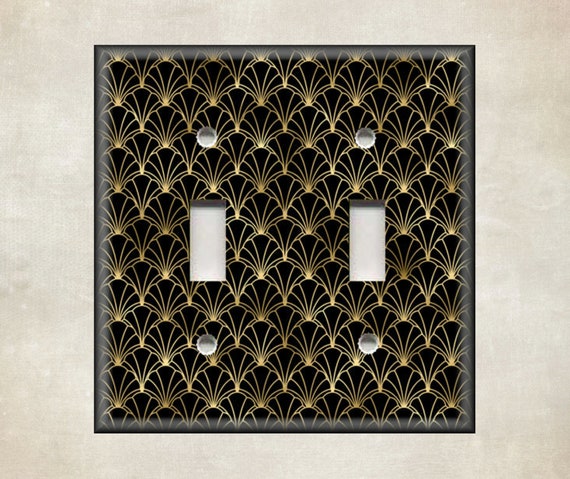The image features an elaborate switch cover plate, possibly made of marble or another white stone. The cover plate encloses a black square inset, adorned with intricate gold patterns resembling a spiderweb, radiating from a central yellow dot and extending vertically in a repeated web-like design. At the center of this black square are two longitudinal white rocker arm switches made from the same material as the surrounding cover plate. Flanking each switch are two dark gray spheres positioned in pairs above and below the rectangular switches, resembling rivets rather than screws, which provides a symmetric and visually appealing accent. The overall design balances functional elements and decorative artistry, resulting in a luxurious and sophisticated appearance.